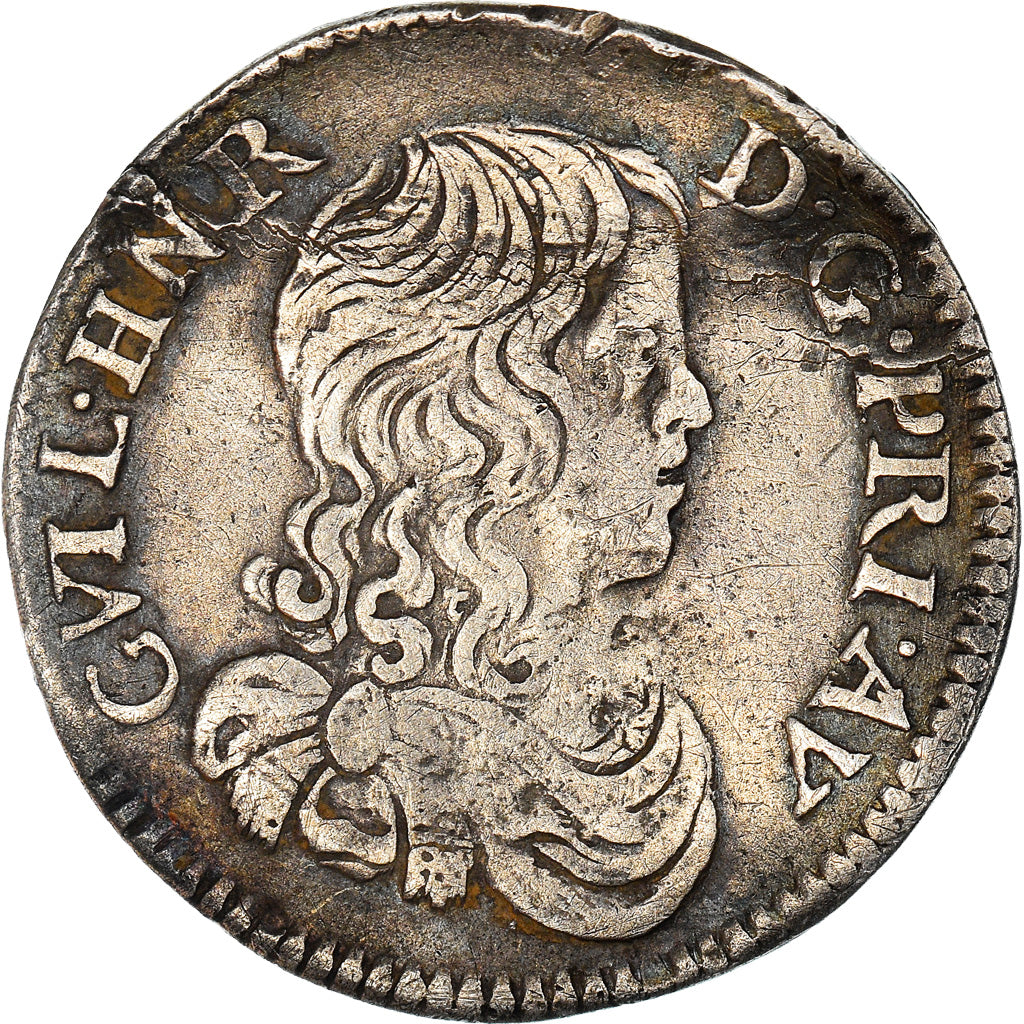This close-up image showcases an ancient, foreign coin sitting on a professional white background, likely intended for sale. The coin, which appears to be metallic and predominantly brown with patches of gray and light brown, features significant wear around the edges. The center of the coin displays an etching of a male figure with long, wavy hair, a hooked nose, and partly open lips, facing to the right. The man is adorned with a distinctive scarf draped around his neck and tied on his right shoulder. The left side of the coin has the characters "G-V-I-L.H-N-R" and the right side displays "D-G.P-R-I.A-V." The outer edge of the coin shows ridging, though some of it is worn away due to extensive use, particularly on the top and left sides. Overall, the intricate details, including the scratches and blemishes, reflect its ancient and dignified history.